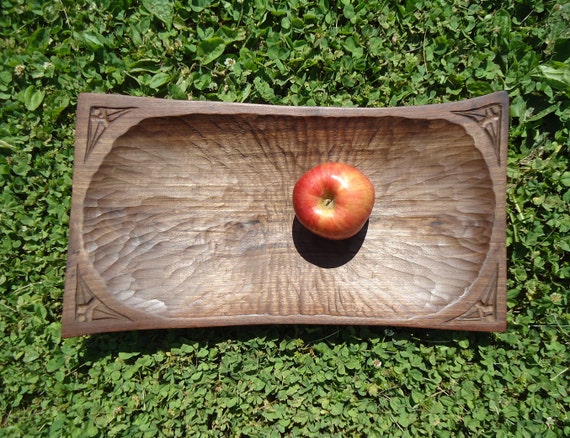In this color photograph taken from above, a single golden red apple sits almost centrally in a somewhat rectangular-shaped, dark brown wooden bowl, positioned amidst a bed of green leafy vegetation, likely low-growing ground cover plants or tiny clovers. The bowl, reflecting sunlight and displaying a lighter gray sheen in some areas, appears hand-carved given its slightly irregular lines. It features an oval-shaped depression in the center with deep gouged grooves, and the corners of its rim are adorned with abstract triangular designs. The apple, resting upright with its stem clearly visible from the top, showcases a light red hue with hints of yellow blush and bright white reflections. A stark shadow underneath the apple indicates bright midday sun, suggesting the photo was taken outside on a sunny day.